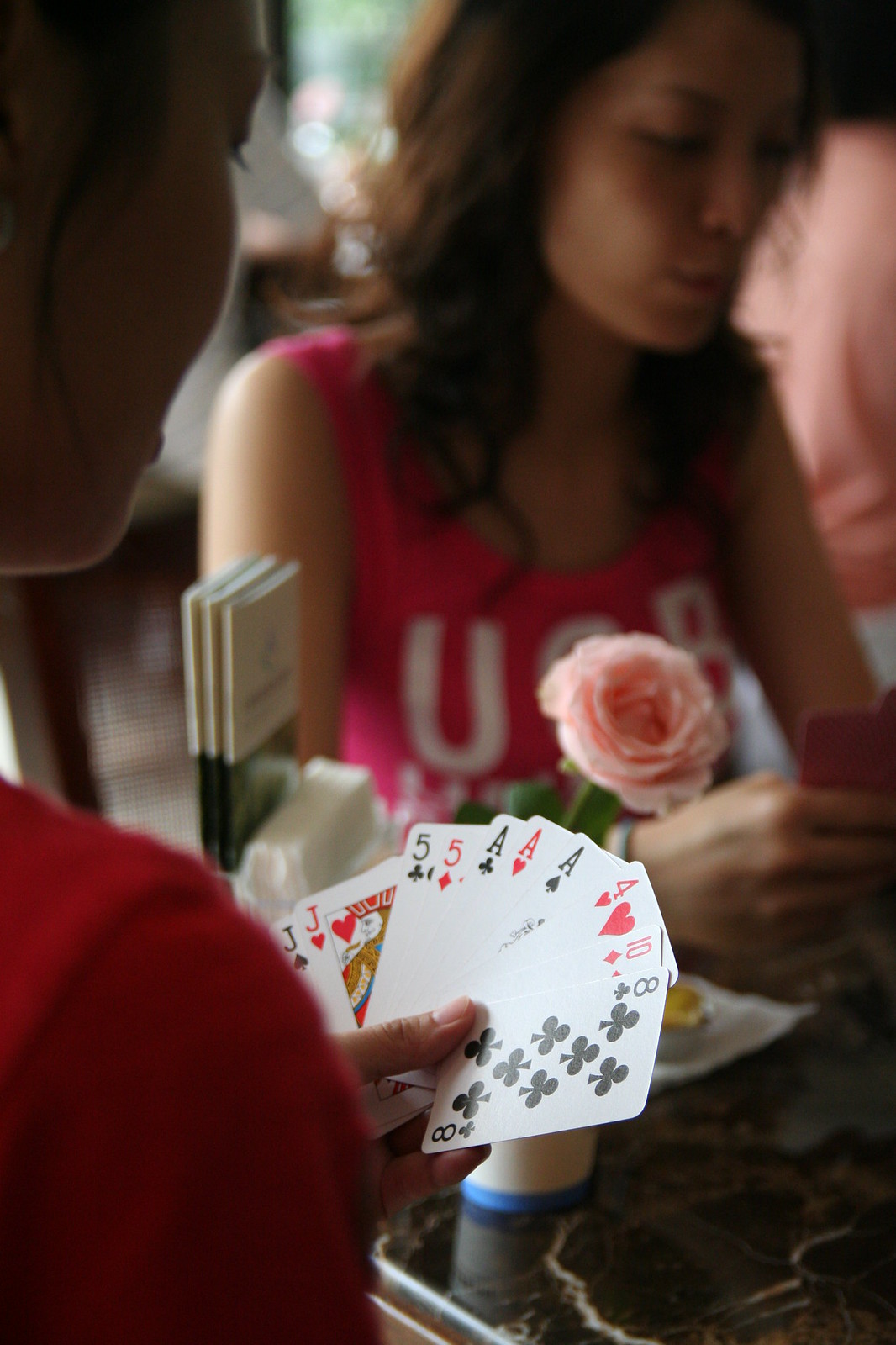In this vibrant photograph, the focal point is two ladies engaged in a lively card game. The lady in the foreground, partially obscured, is seen in a red shirt, with part of her side profile visible. She is intently holding a diverse hand of cards, including the eight of clubs, ten of diamonds, four of hearts, ace of spades, ace of hearts, ace of clubs, five of diamonds, five of clubs, jack of hearts, and jack of spades. A single strand of her hair delicately traces her cheek, as her hair is neatly tied up. On their table, with its distinct tortoiseshell finish, a vase housing a pink rose adds a touch of elegance. Also present on the table is a holder containing various pamphlets. The opposing player, a lady with flowing dark hair cascading to her shoulders, wears a pink tank top adorned with the visible letters 'U' and 'B'. She holds a set of playing cards with red backs. In the background, sunlight streams into the room, casting a warm glow over additional objects, one of which is a seated individual just beyond the engaged players, adding depth and life to the scene.